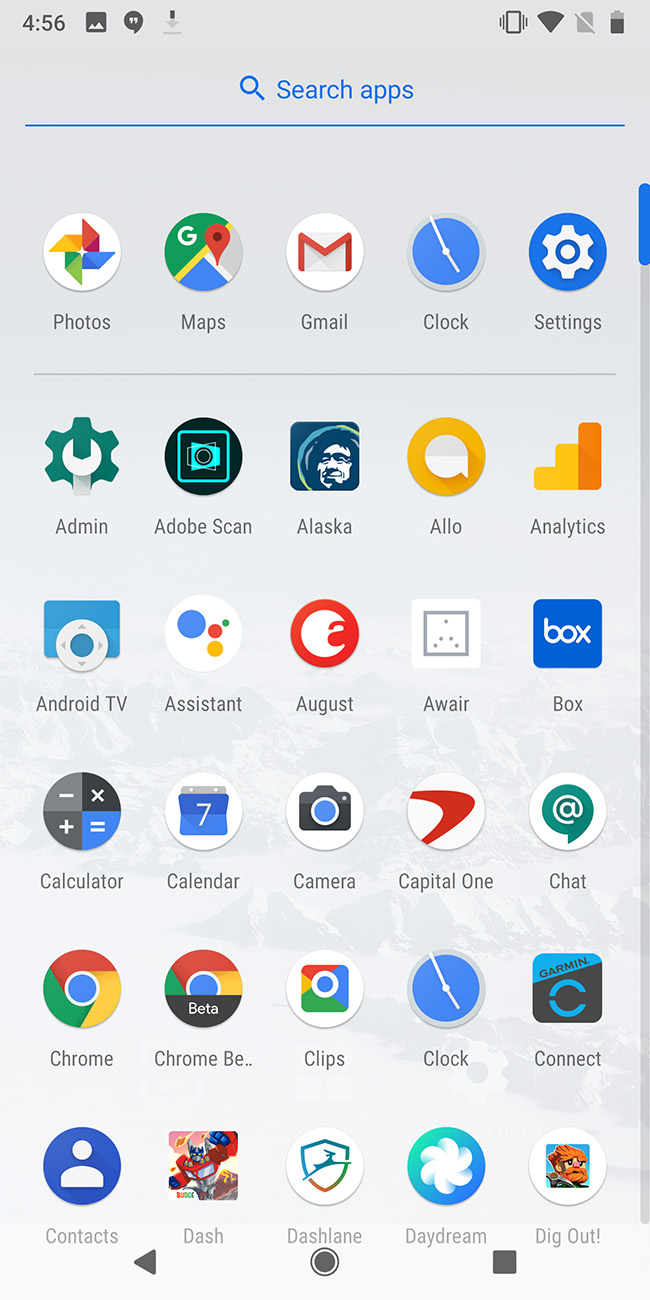The image displays a user interface with a light blue background. At the top, the number "456" is prominently shown along with several icons. Below this, there is a search bar featuring a small blue magnifying glass icon. A thin blue line separates the search bar from the next section. This area includes icons for various applications such as Photos, Maps, Gmail, Clock, and Settings. On the far right is a blue slider bar.

Below this, there is an extensive list of application icons, including Admin, Adobe Scan, Alaska, Allo, Analytics, Android TV, Assistant, August, Aware, Inbox, Calculator, Calendar, Camera, Capital One, Chat, Chrome, Chrome Beta, Clips, Clock, Connect, Contacts, Desk, Desktop, Daydream, and Dig Out. At the very bottom of the image, there are three navigation icons: a black triangle, a black circle, and a black square.